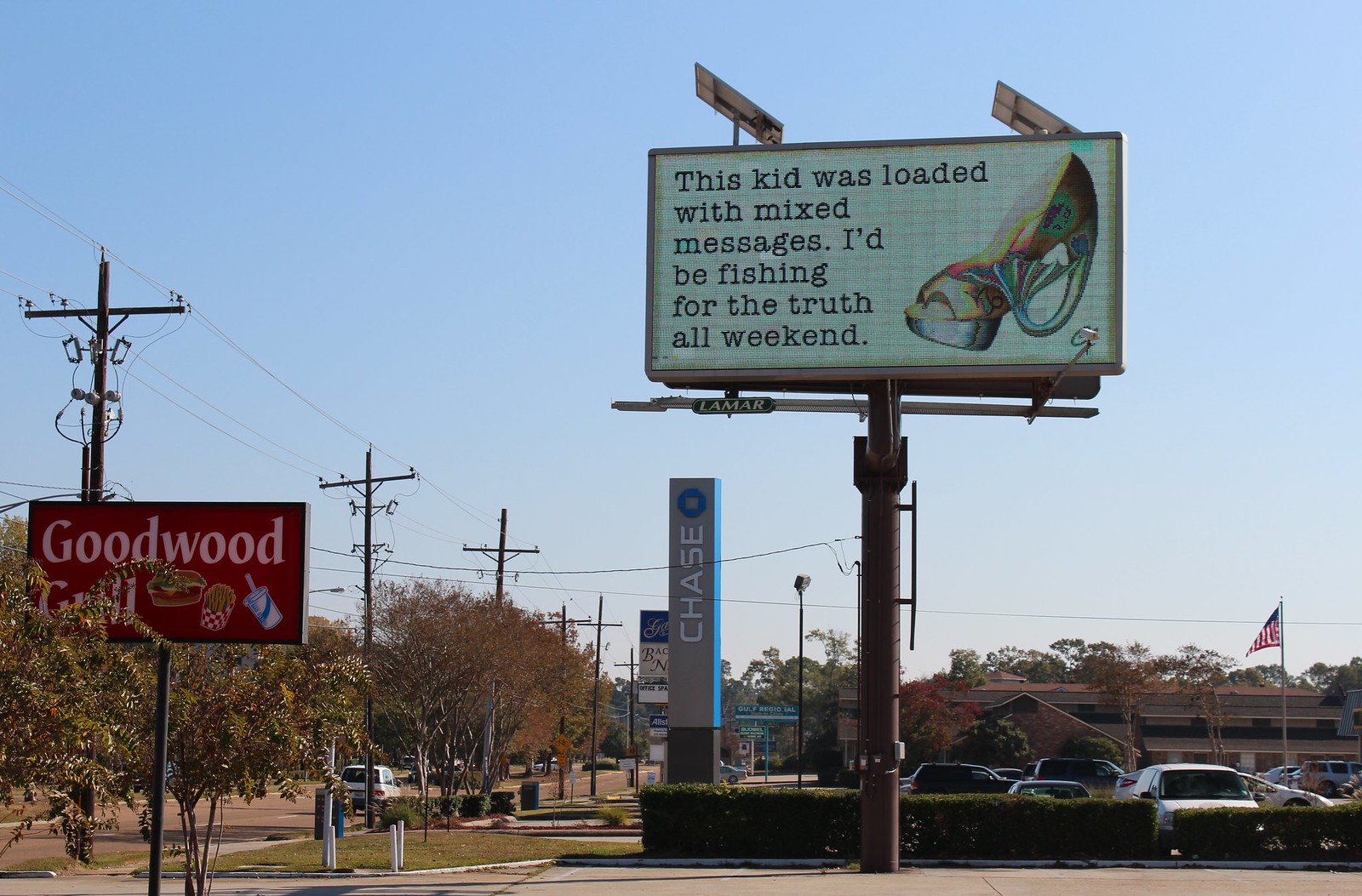The photograph captures a bright, clear day with a vivid blue sky. On the left side of the image, utility power lines weave through a cluster of leafy green and brown-orange trees. Prominently displayed is a red billboard advertising "Goodwood Grill" in bold white font, featuring a visually enticing image of a burger and fries in a cup.

To the right side of the composition, there stands a tall, gray structure labeled with the word "Chase" in white letters accompanied by a blue circle, representing the well-known bank. Near this structure, another large billboard, mounted on a metal pole, features a stark white background with dark text reading: "This kid was loaded with mixed messages. I'd be fishing for the truth all weekend." 

Adjacent to this billboard, an intriguing, shoe-shaped object with a fish fin – a multicolored creation in hues of yellow, red, blue, and green – adds an element of whimsy to the scene.

Below these focal points lies a parking lot with several cars, in front of a tan and brown building in the background. Standing tall and proud in the scene is an American flag on a flagpole, billowing gently in the breeze.